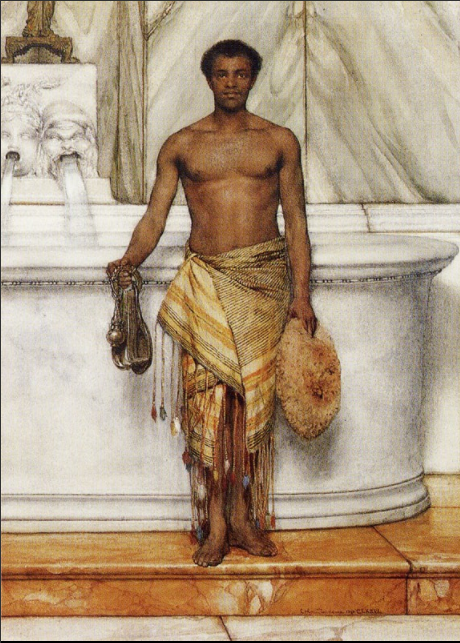The semi-realistic artwork depicts a tall African man standing in a large, marble bathhouse. He is shirtless and wears a tribal sarong adorned with red, blue, and white tassels, which is tied at the waist. The floor beneath him is a striking reddish-brown and white marble, while the walls are composed of pristine white and black marble. In front of him stands an imposing, waist-high white tub, into which water is being poured from the mouths of two stone faces—one appearing angry, the other frightened. In his right hand, the man holds an intricate device with a ball and what seem to be ropes or pulleys. His left hand grips a large, round object that could either be a hat or a giant sponge. The detailed scene captures the serene yet intense ambiance of the bathhouse.